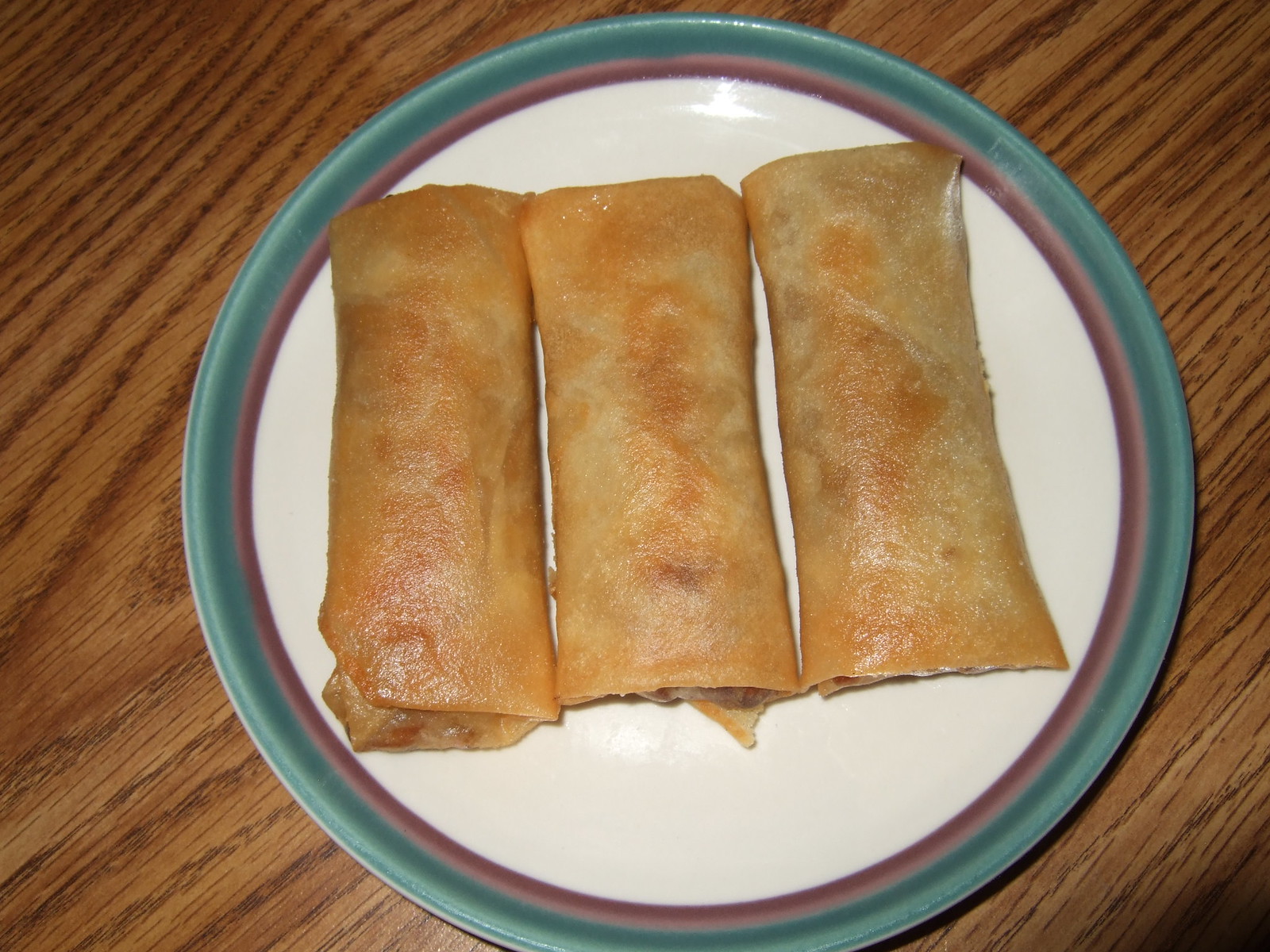This vibrant color photograph captures three beautifully arranged spring rolls that appear to be sausage-filled. They are golden-brown with hints of gloss and a slightly crisp texture, indicative of deep frying or baking, revealing some of the ingredients beneath their shiny surface. The rolls are positioned in the center of a round, off-white ceramic plate. The plate features a decorative perimeter, transitioning from a thin reddish-brown strip to a jade and light green outer rim. The background of the image showcases a synthetic wooden surface in varying shades of brown, adding warmth to the overall composition. The lighting is bright, likely from a camera flash, enhancing the vividness of the colors and details. The meticulous arrangement and the harmonious blend of hues present a visually appealing and appetizing tableau.